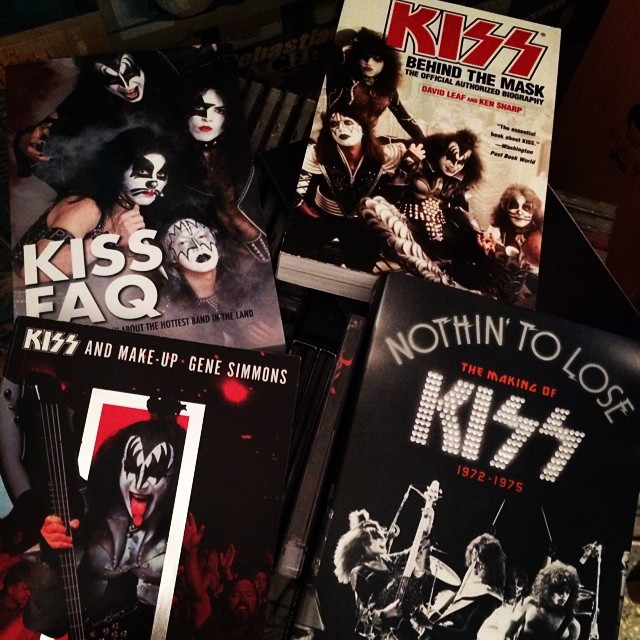This image showcases a collection of KISS memorabilia neatly arranged on a black table. Prominently featured is a book titled "Nothing to Lose: The Making of KISS, 1972-1975" with a black cover and white letters, depicting the band members, including one playing guitar and another on the drums. To the left, a striking image of Gene Simmons with his signature long tongue, white face paint, and black eye makeup is seen on the cover of "KISS and Makeup." The "KISS FAQ" book, displaying the faces of all four band members in their iconic makeup, sits above it. The top of the arrangement shows "KISS: Behind the Mask," a white-covered book with red print, credited as the official authorized biography by David Leif and Ken Sharp. This comprehensive display reflects the vibrant history and enduring fan interest in the legendary rock band KISS.